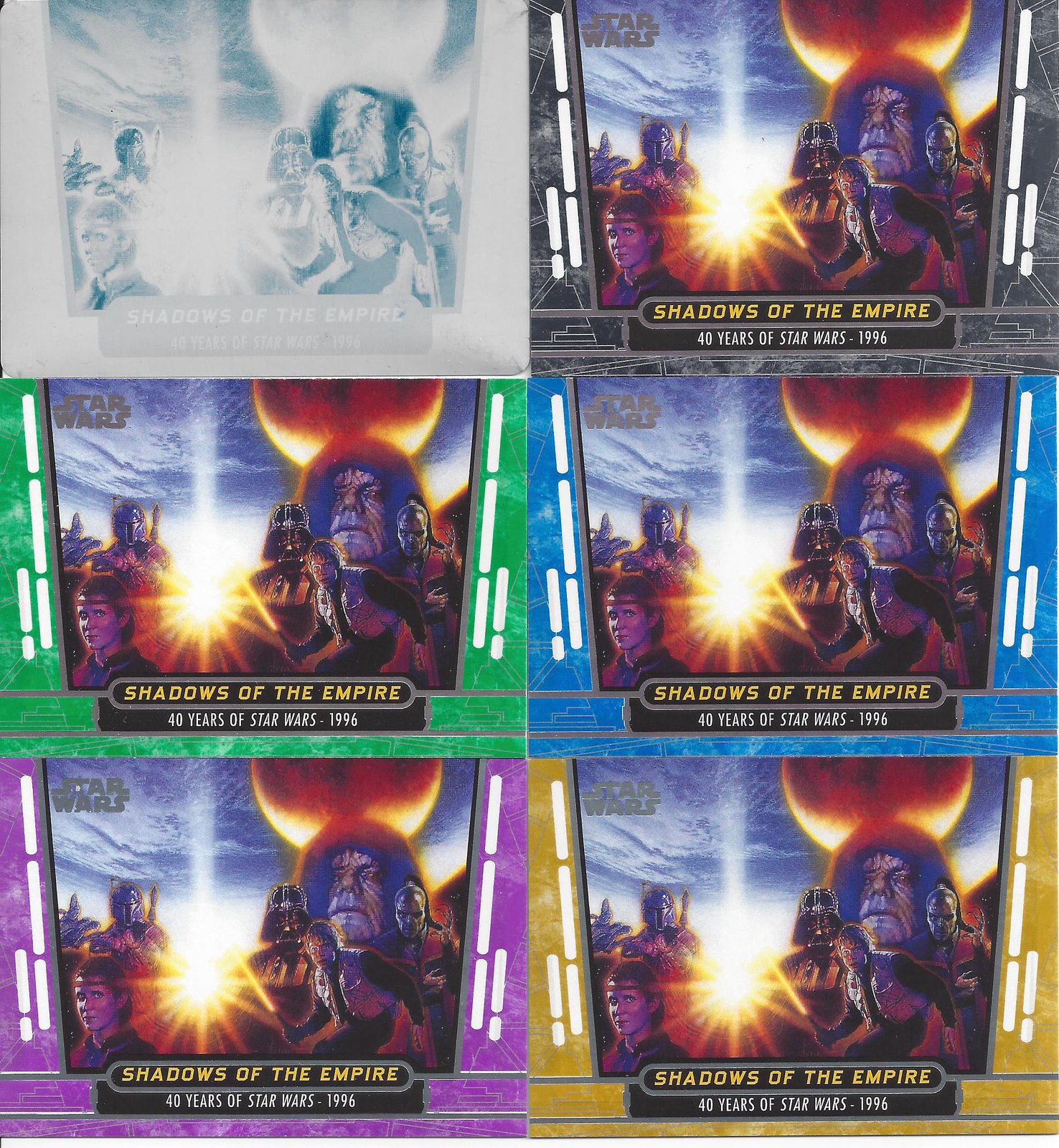The image is a collage of six Star Wars-themed trading cards arranged in two columns of three rows. Each card features the same artwork but with varying border colors: white (top left), green (middle left), purple (bottom left), gray (top right), blue (middle right), and yellow (bottom right). The central image showcases prominent Star Wars characters, including Darth Vader and Boba Fett on the left side, with the Emperor located towards the right side. In the background, there is a depiction of Earth and a red planet. Each card prominently displays the text "Shadows of the Empire" in yellow at the top, and below that, "40 Years of Star Wars, 1996" in white.